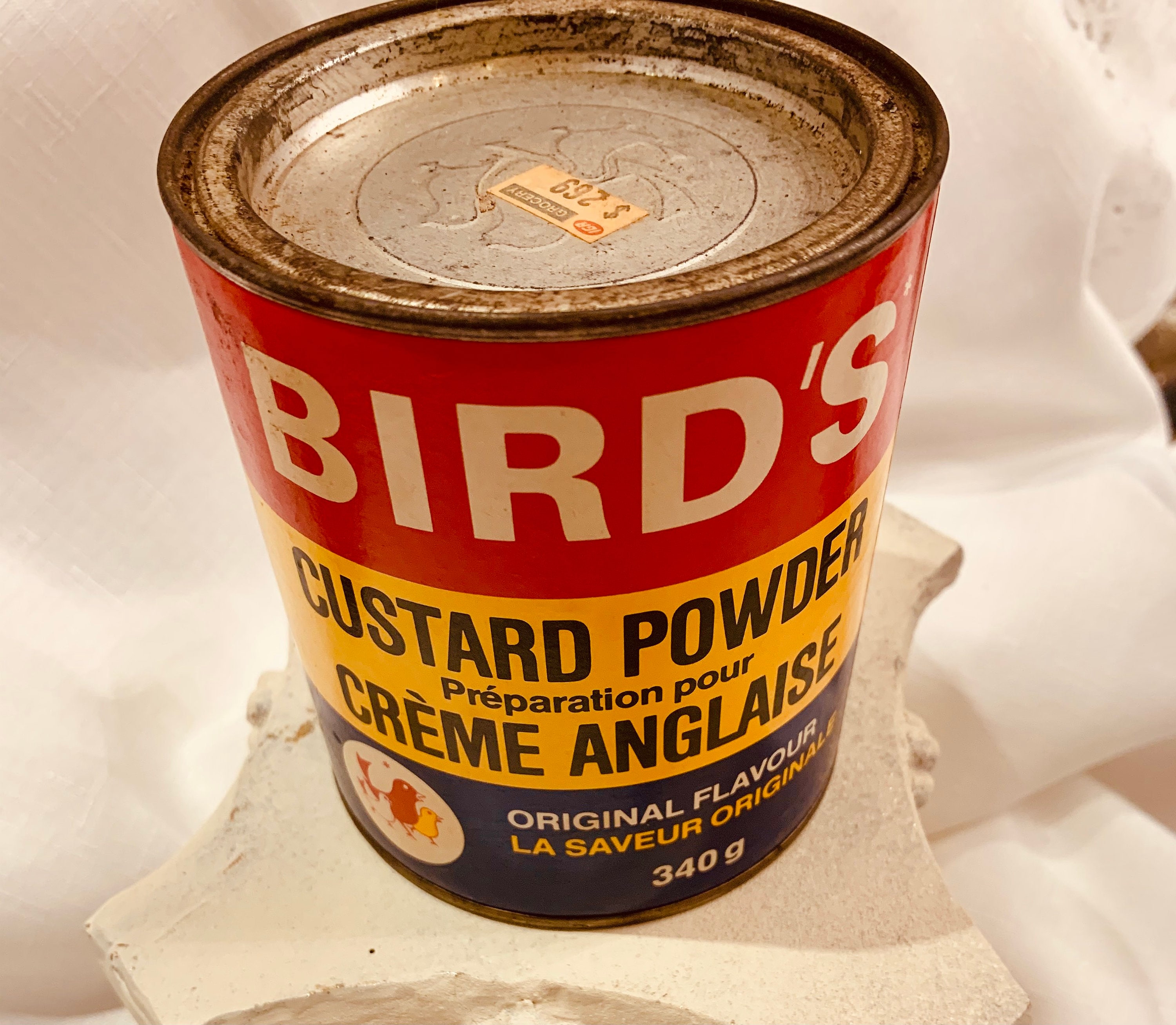The image showcases an old, rusty can of Byrd's custard powder, prominently displaying age-related wear with significant rust on the lid and bottom. The can is cylindrical, approximately the size of a tobacco tin, featuring a pry-off lid that sits heavily rusted and appears to have a price tag of $2.69. The can is adorned with a tri-colored label in red, yellow, and blue, which divides the content into sections. The red top section displays 'Bird's' in bold white letters. Below, the yellow section has 'custard powder preparation pour crème anglaise' written in black text, indicative of an English cream preparation. The bottom blue section features a white circle containing a red and yellow chicken logo, accompanied by the phrases 'original flavor' and 'la saveur originale,' denoting its original taste, and includes a weight specification of 340 grams. The can is placed on what appears to be a piece of white stone, partially covered by a white cloth.